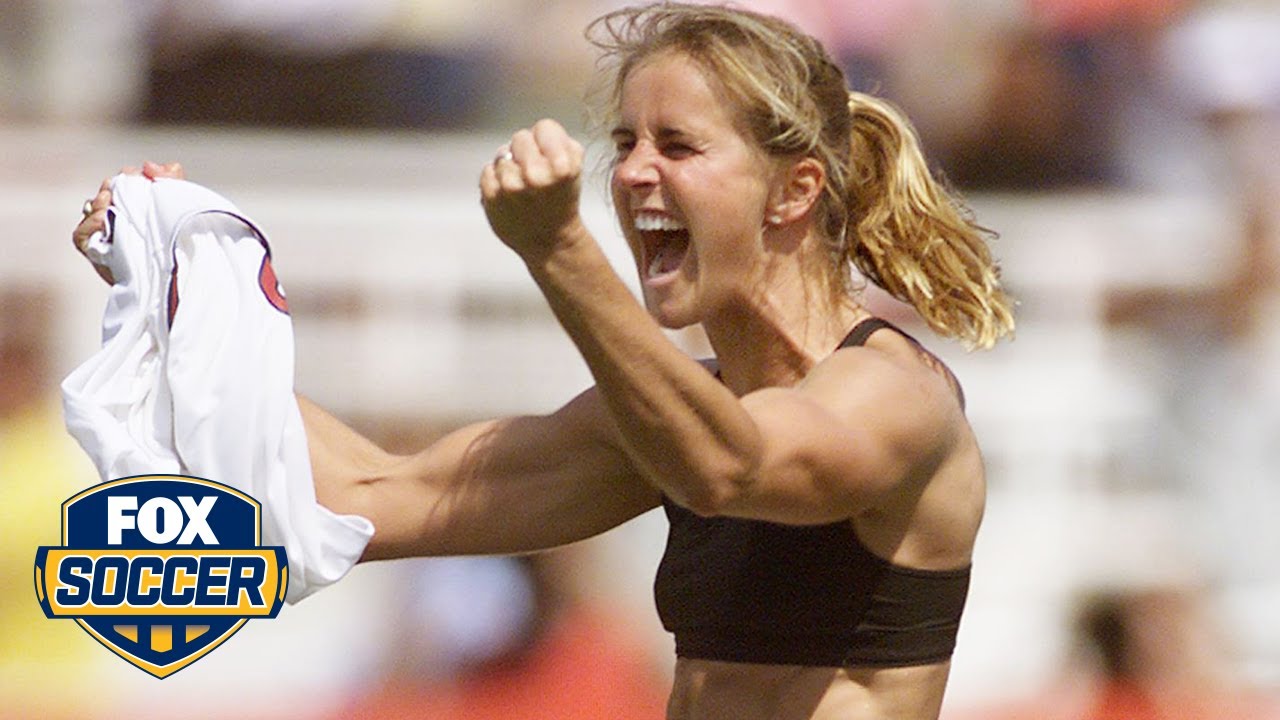This photograph captures a triumphant moment of a female soccer player celebrating during a sporting event. The focus of the image is a young Caucasian woman, likely in her late 20s to early 30s, characterized by her muscular build and pronounced biceps, indicative of a professional athlete. She has blonde hair tied in a ponytail, accentuating her energetic demeanor. The woman is positioned centrally, looking towards the left in a semi-profile view, her face radiating sheer joy with her mouth wide open and eyes nearly closed as she shouts in celebration. 

She victoriously holds her white jersey with red lettering in her right hand, having just removed it to reveal a brown sports bra with racerback straps underneath. Both her arms are raised, fists clenched in a powerful gesture. The background features a blurred, bokeh effect that hints at a sporting stadium filled with vibrant activity, though these elements are out of focus to emphasize her ecstatic moment. 

In addition to her jubilant posture, she wears silver rings on both ring fingers, adding a subtle touch of personal style. The image prominently features a logo in the bottom left corner that reads "Fox Soccer," indicating that this momentous occasion was likely broadcasted on the Fox channel for a wide audience, presumably after she scored a decisive goal.